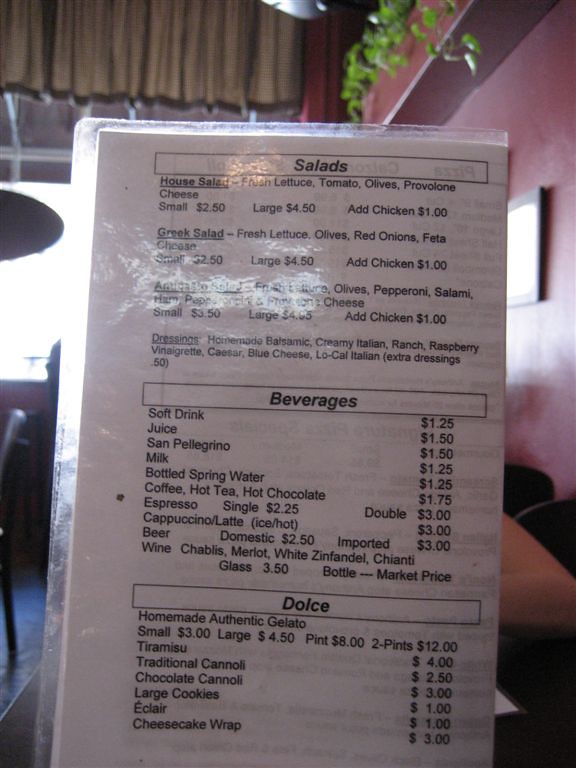The image captures the intimate, cozy atmosphere of a doner restaurant, focusing closely on a laminated white menu with black text. The menu, which constitutes three-fourths of the image, is straightforward with sections for salads, beverages, and desserts, though a glare on the lamination slightly obscures the text. At the top, salads like House Salad and Greek Salad are listed with various dressings and sizes. The middle section features beverages, including soft drinks, San Pellegrino, coffee, and alcoholic options like beer and wine. The bottom section, labeled "Dulce," offers sweet treats such as homemade gelato, tiramisu, cannoli, and eclairs.

Along the left edge and top of the menu, the lamination extends slightly beyond the paper. The right side of the image reveals a person’s bent left elbow, suggesting they are seated at the table across from the menu holder. The backdrop includes a warm pink wall adorned with a shelf, a single central picture, and a hanging pothos plant in the top right corner. Left of the menu, sunlight streams through the establishment’s window, hinting at a bright day. Part of a chair's back is also visible on this side, but the menu largely dominates the view, creating a sense of an inviting yet detailed setting for a meal.